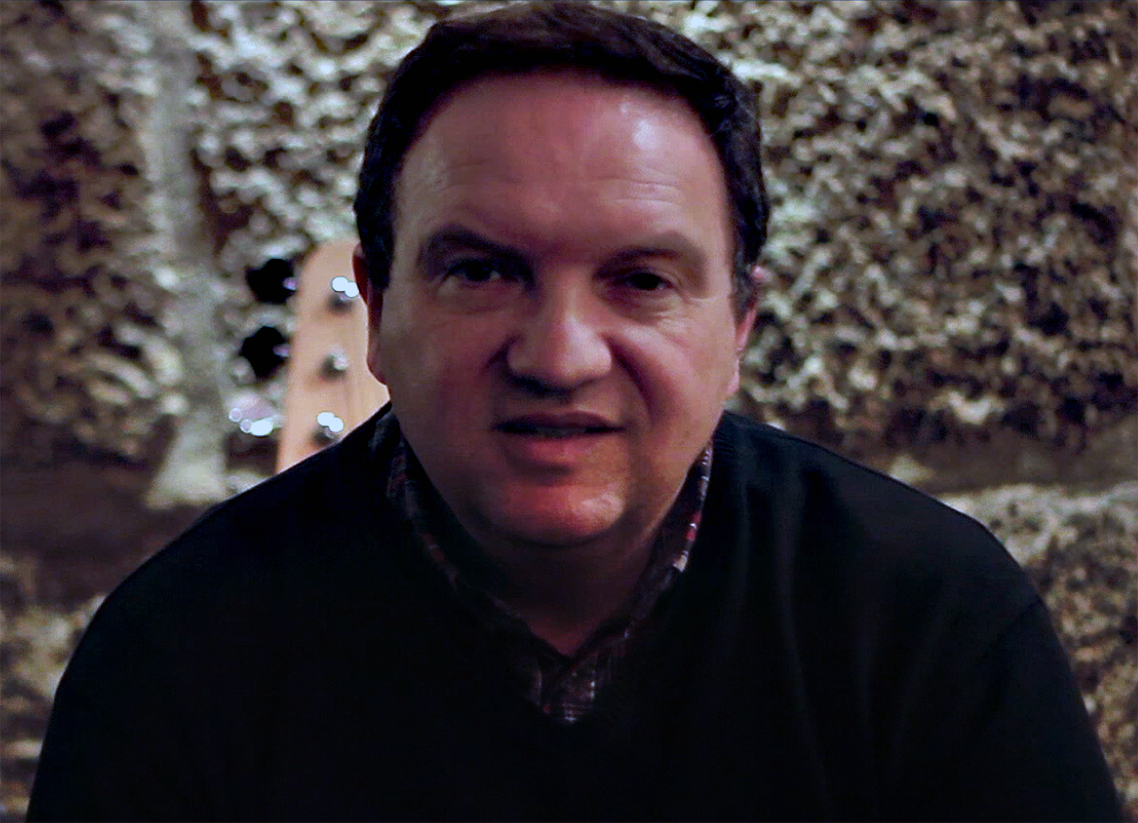This photograph is a portrait of an older white gentleman seated and facing the camera. He has a plump face and figure, with short brown hair that is slightly receding at the top. The man is dressed in a black sweater, under which a plaid dress shirt is peeking through at the collar. His expression is one of a half-smile, possibly captured mid-speech. Wrinkles adorn his face, hinting at his age. The lighting in the image creates a contrast, with the right side of his face more illuminated than the left. Behind him, a musical instrument, likely a guitar or bass, can be seen peeking out. The background is a rough, stone-like texture with a small light source above, adding warmth to the scene. Additionally, a table can be discerned on the left side of the image, partially visible. Overall, the photo focuses intently on the man's face and upper torso, providing a detailed and intimate portrayal against the softly blurred backdrop.